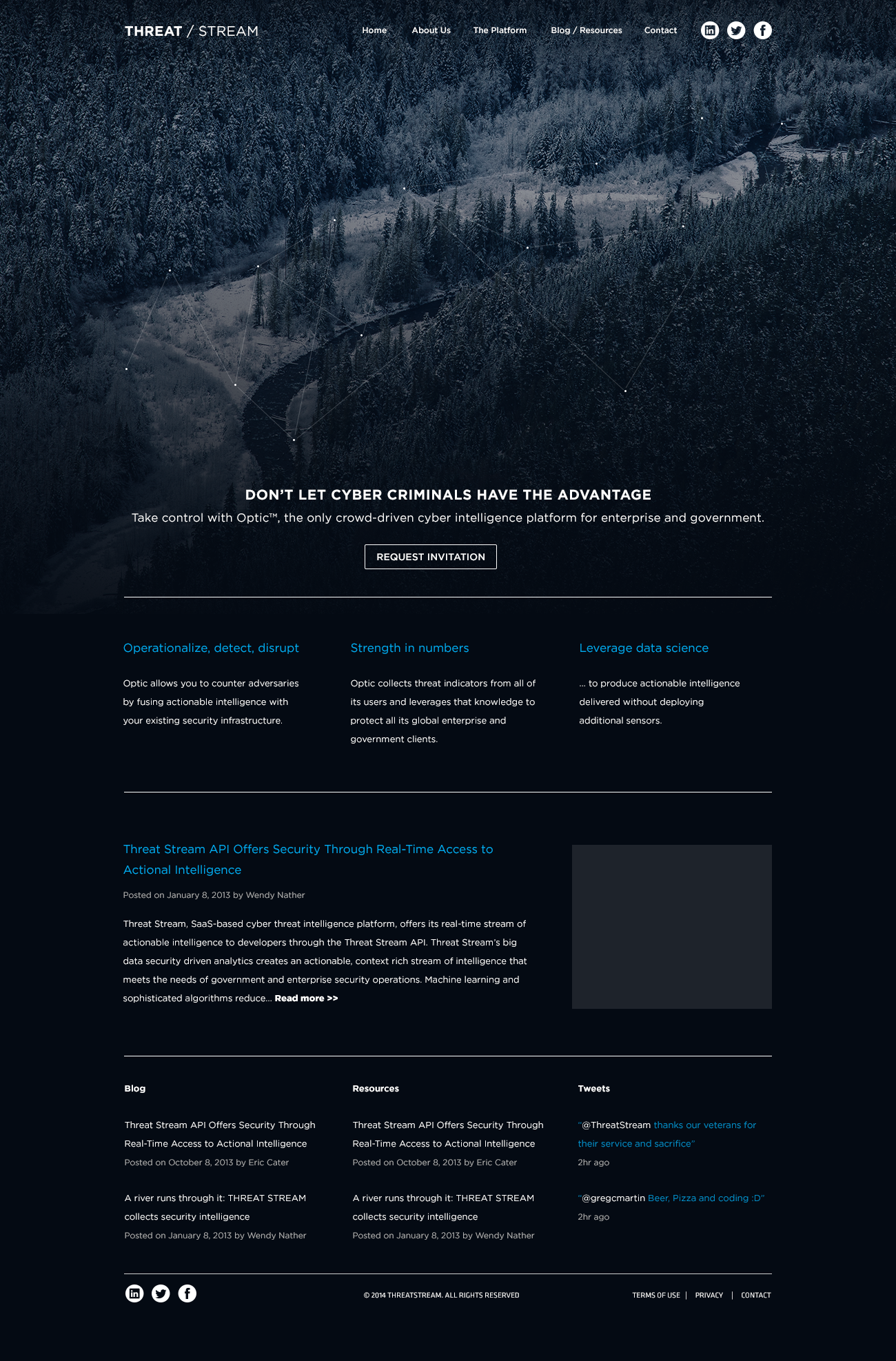In the image, a sophisticated digital landscape is depicted, featuring interconnected data points illustrated by lines and dots overlaid on a block of resources, with trees serving as the background. The main focus is a bold text that reads: "Don't let cybercrime take the advantage. Take control with Optic, the only product-driven cyber intelligence platform for enterprise and government. Request a demonstration."

Beneath this, a tagline emphasizes the operational effectiveness: "Operationalize your cyber defense. Optic allows you to counter adversaries by fusing actionable intelligence with your existing systems."

The description further elaborates that Optic aggregates indicators from all its users into a cohesive knowledge project, which benefits global enterprises and government clients. It employs data science to produce actionable intelligence without the need for additional sensors, enhancing current operational frameworks. The platform offers an API that provides access to national intelligence threat streams, creating a hybrid solution backed by potent data insights and real-time intelligence.

The image concludes by highlighting Optic’s commitment to delivering quality intelligence, fostering a collaborative defense strategy against cyber threats.